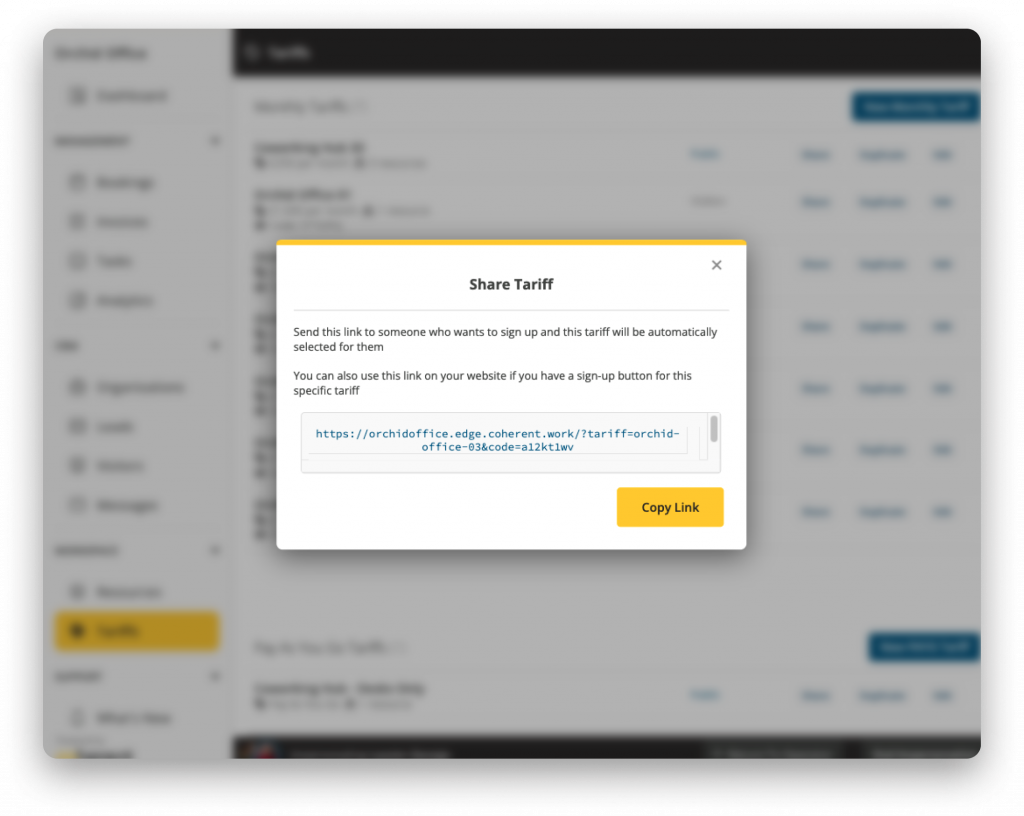A blurred webpage filled with dense, complicated-looking technical information serves as the backdrop. A prominent, in-focus pop-up dialog box titled "Share Tariff" dominates the foreground. The message within the pop-up instructs users to send a provided long URL to individuals interested in signing up, automatically selecting the specified tariff for them. It also suggests using the link on a website's sign-up button for the particular tariff. Below the URL is a "Copy Link" button. The blurred background reveals a white interface with several panels displaying black text, interspersed with blue elements like links and buttons, hinting at a detailed and possibly intricate web-based application.